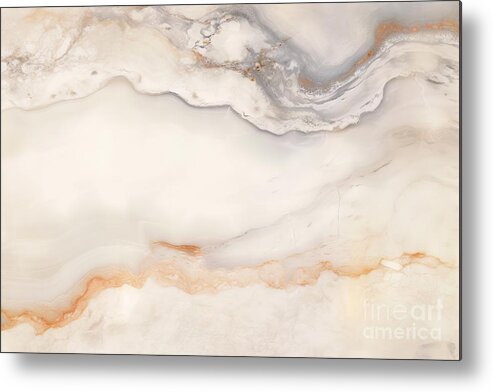This image features a photograph of an abstract painting displayed against a white background, capturing an outdoor setting. The painting, presented with a slight 3D effect due to its tilted angle and the visible shadows along its right side, depicts a marbled surface with an array of cream, gray, and orange bands. The artwork's texture and pattern evoke the appearance of rock sediment. Notably, an orange wavy band near the bottom runs across the painting, ending in a slight downward curve. Above this, a series of white and gray wavy bands mirror the contour of the orange band below. The symmetrical design is further enhanced by a brown wave mimicking the orange wave's shape. The painting's edges are gray or black, adding a subtle border. In the bottom right corner, there is a watermark that reads "Fine Art America," the sole text present on the painting.